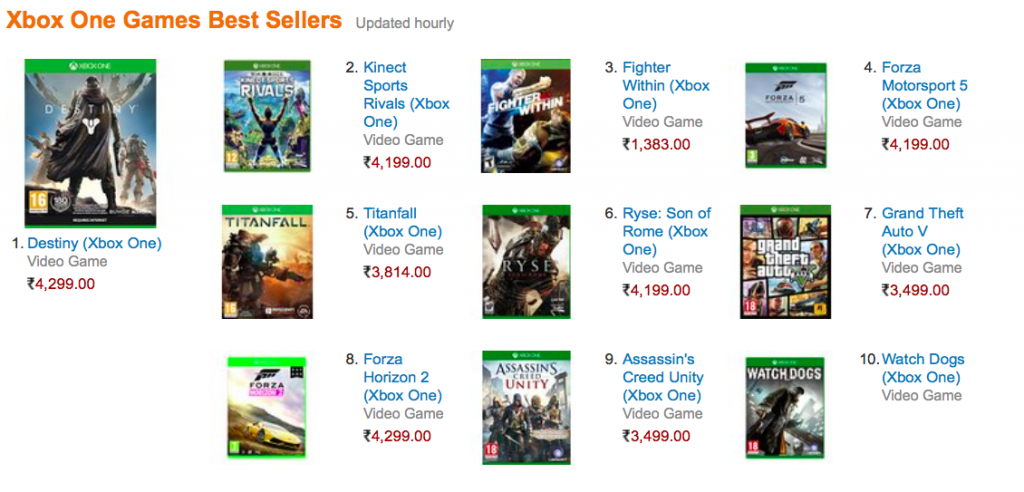The image is a screenshot of a web page featuring a list of the best-selling Xbox One games, presented on a white background. The image is horizontally oriented, with approximate dimensions suggesting a wide rectangular shape. 

In the top left corner, the text "Xbox One Games Best Sellers" is displayed in orange, followed by a note indicating the rankings are updated hourly. 

On the left side of the image, there is a thumbnail of the game "Destiny" for Xbox One. Below the thumbnail, "Destiny Xbox One" is written in blue text, followed by the words "Video Game" in gray. The price is marked in red text as $42.99.

The list of the top ten best-selling games, arranged from top to bottom and left to right, includes:

1. **Destiny Xbox One**
   - Price: $42.99

2. **Kinect Sports Rivals Xbox One**
   - Price: $41.99

3. **Fighter Within Xbox One**
   - Price: $13.83

4. **Forza Motorsport 5 Xbox One**
   - Price: $41.99

5. **Titanfall Xbox One**
   - Price: $38.14

6. **Rise Son of Rome Xbox One**
   - Price: $41.99

7. **Grand Theft Auto V Xbox One**
   - Price: $34.99

8. **Forza Horizon 2 Xbox One**
   - Price: $42.99

9. **Assassin's Creed Unity Xbox One**
   - Price: $34.99

10. **Watch Dogs Xbox One**
   - (Price not given in the original description)